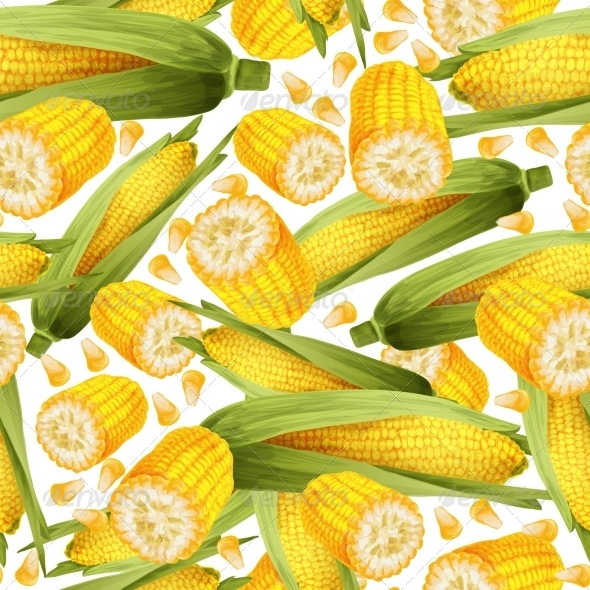The image features an illustration of corn in various stages, all floating against a bright white background. The scene is filled with a multitude of corn cobs, including whole ones still wrapped in their vibrant green husks and others fully exposed. Additionally, there are corn cobs meticulously cut into sections, prepared as if for cooking, revealing the vivid yellow and white ends. Scattered throughout the composition are individual corn kernels, mostly yellow with some white tips, adding to the diverse display. The overall effect is a vibrant, almost painting-like depiction, emphasizing the mix of colors and textures in a seemingly floating arrangement of corn.